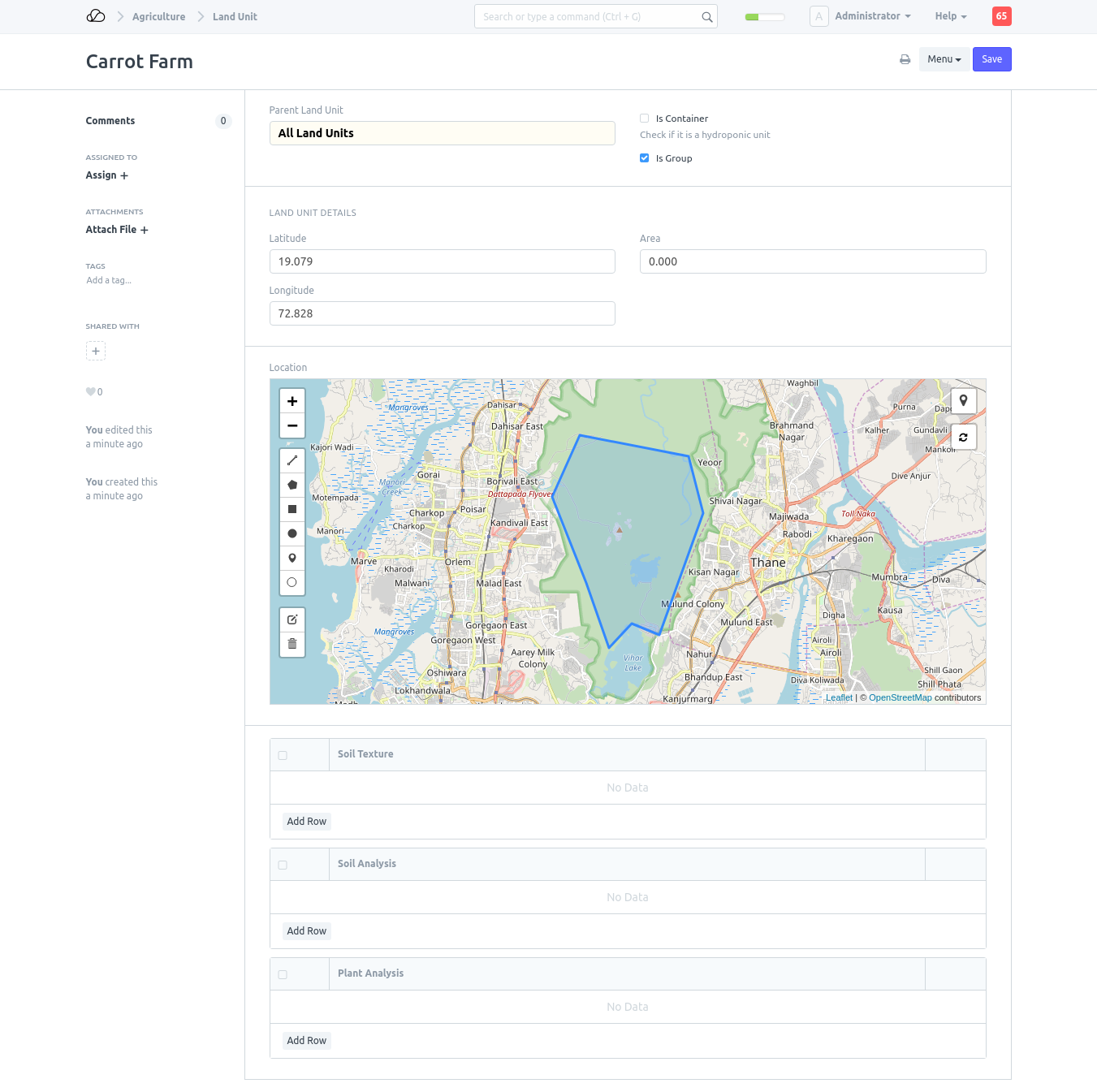This screenshot captures a webpage from an unidentified website dedicated to agricultural land management. At the top, a thin gray banner features navigation options: "Agriculture," "Land Unit," "Search or Type a Command," "Administrator," and "Help." Below this banner, the page is titled "Carrot Farm."

On the left side of the screen, a vertical menu provides various interactive options, including "Comments," "Assign to," "Attachments," "Attach File," "Tags," "Add a Tag," and "Shared With." A brief note indicates recent user activity: "You edited this a minute ago," and "You created this a minute ago."

To the right, additional sections include "Parent Land Unit" and "All Land Units." A checkbox labeled "Is Container, check if it is a hydroponic unit" remains unchecked. However, another checkbox, "Is Group," is marked as checked.

Further down, within the "Land Unit Details," the geographical coordinates are listed as Latitude 19.079 and Longitude 72.828, with an area measurement of 0.000. The "Location" field features an embedded map with a highlighted central area, though the map's specific location remains uncertain. 

Below the map, various fields display placeholders with no current data, including "Soil Texture," "Soil Analysis," and "Plant Analysis," each accompanied by an "Add Row" option for future inputs.

The screenshot includes no people, animals, or automobiles, emphasizing a purely functional and data-oriented interface.